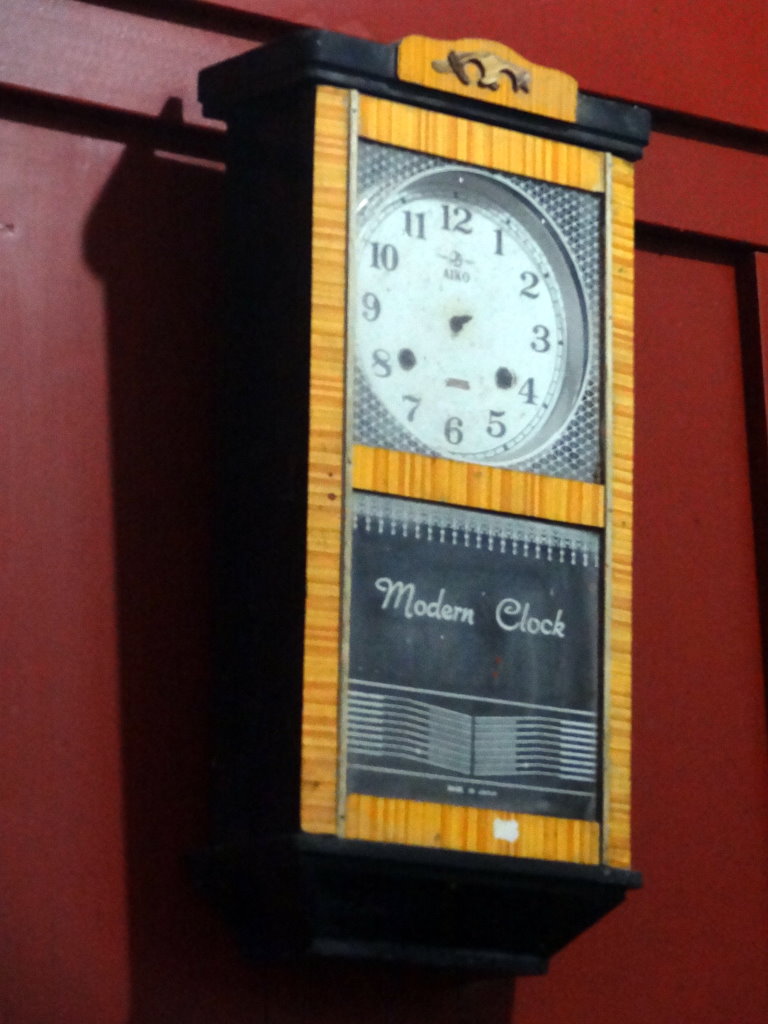A modern clock is mounted against a bold red wall, accentuating its striking design. Nearby, there appears to be a structure resembling a red bed frame. The clock itself intriguing and enigmatic, lacks traditional hands and instead features two dots, suggesting a unique time-telling mechanism. Below the clock face, subtle lines reminiscent of vintage radio dials add a touch of nostalgia. Although there are small, indecipherable words at the bottom, their meaning remains elusive even upon close inspection. At the top of the clock, a familiar decorative element reminiscent of those found on grandfather clocks further enhances its vintage charm, blending the old with the contemporary in a visually captivating manner.